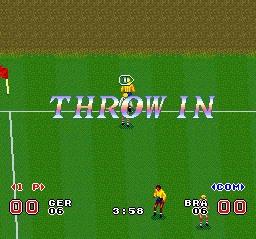This image is a snapshot from a soccer video game. In the foreground, the text "Throw In" is prominently displayed, indicating that a throw-in is about to take place. Behind these words, a player is standing just off the field, preparing to throw the ball back into play. Another player stands in bounds, ready to receive the ball. Two additional players are visible in the bottom right corner of the screen. 

The score is clearly depicted by two red zeros situated in the bottom corners—one in the bottom right and one in the bottom left—indicating that both teams are tied at 0-0. The game clock at the bottom center of the screen shows 3 minutes and 58 seconds, along with additional game statistics nearby. The soccer field is a vibrant green, patterned with alternating light and dark green stripes. Beyond the field, the ground changes to a yellow-brown hue, contrasting with the lush playing surface.